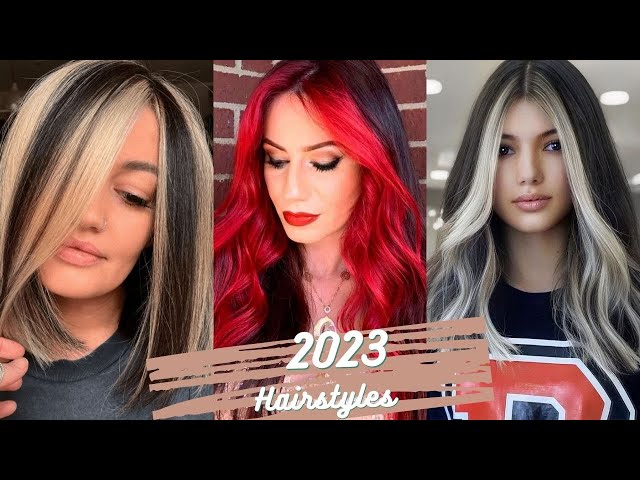This image appears to be a YouTube thumbnail advertising popular 2023 hairstyles. The thumbnail features three distinct images of women, possibly the same woman with three different hairstyles, arranged to fill the space of a widescreen format. 

At the bottom center of the thumbnail, there is text that reads "2023 Hairstyles" in yellow or white, set against an orangish-red background for emphasis. The top and bottom borders of the entire image are black, framing the pictures neatly.

The leftmost image shows a woman who seems to be in her thirties with brown and blonde streaks alternating through her hair. Her hairstyle showcases sections of both black and blonde strands, and she is wearing noticeable lipstick.

In the middle image, the woman has striking hair with a vibrant red front and a brunette back. She also sports red lipstick and the color contrast in her hair and makeup is quite eye-catching.

The rightmost image features a woman with brunette hair accented by blonde highlights near her face. Her hair is parted directly in the middle, and she is wearing a black shirt. Her hair, with its frontal blonde streaks, falls across part of her face but still reveals her brown eyes, nose, and mouth. She is described as young-looking.

Overall, the thumbnail effectively showcases three varied and trendy hairstyles for 2023, emphasizing bold color contrasts and modern styling techniques.